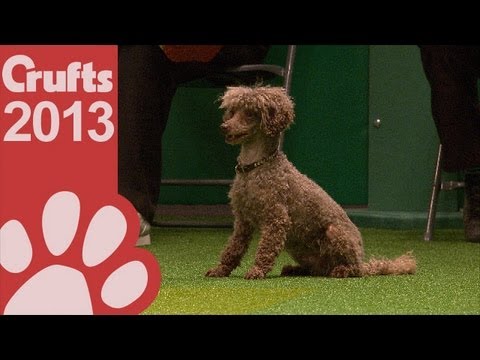The image features a brown, fluffy poodle-type dog with curly, short hair, except for its head, which sports longer hair resembling a bob cut. The dog is sitting on lime-green Astroturf and facing to the left, with its mouth slightly open and wearing a collar. Its tail is medium-length and also curly. The backdrop includes a green wall and the partial view of chairs and a person’s leg. The picture is horizontally aligned with thick black borders on the top and the bottom. On the left side, there is a distinct red rectangular border containing the text “Crufts 2013” in white, accompanied by a white paw print icon.